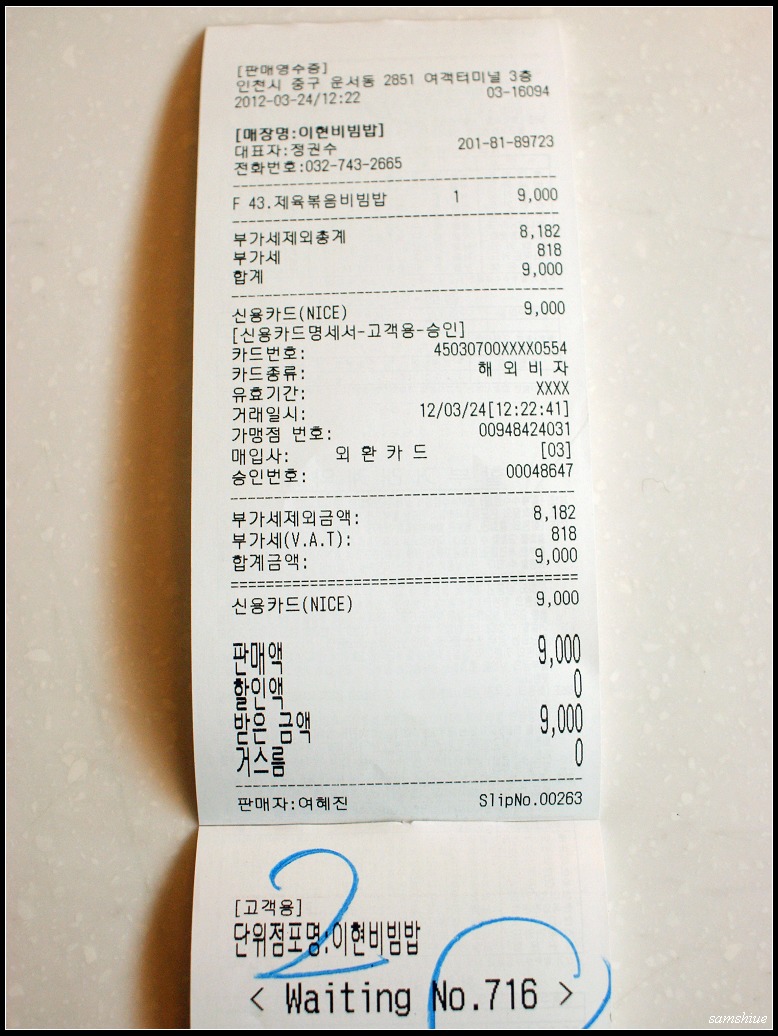This image depicts a printed-out receipt, lying on a slightly speckled white tabletop surface. The receipt is entirely in Hangul, indicating it's in Korean. The text is arranged in columns on the left side, while the right side displays various numbers, likely prices, with some values reaching as high as 9,000. The receipt has a shadow to its left and is attached at the bottom to a second receipt, on which the number "2" is prominently written in blue pen, possibly alongside a "0" or a circled figure. At the bottom of the image, the only English text is visible, stating "Waiting Number 716," with arrows pointing on either side of the number and text.